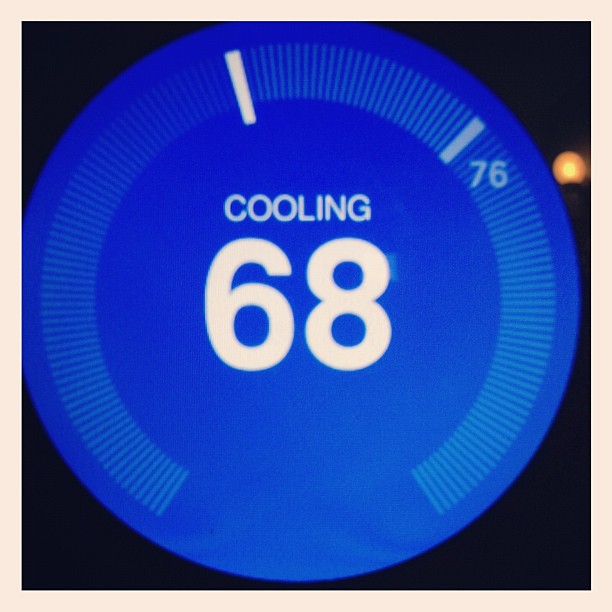The image depicts a square photograph with a black background. Positioned in the upper right third of the frame, there is a small orange circle that contains a smaller yellow circle within it, the function of which is unclear. Dominating the center of the black square is a large, medium-blue circle. In the center of the blue circle, the number "68" in white stands out prominently, with the word "cooling" displayed above it, suggesting that this image is of a thermostat or a temperature display.

Encircling the interior perimeter of the blue circle, except for the bottom eighth portion, is a series of uniformly spaced, small white lines, likely serving as temperature indicators. Approximately a third of the way up these lines, there is a thicker white line marked with "76" beneath it. About a quarter of the way through these lines, a slightly darker white line extends downward, presumably indicating the current temperature of 68 degrees. Beyond this marker, the series of uniform white lines continue around the circle until the unfinished section at the bottom.